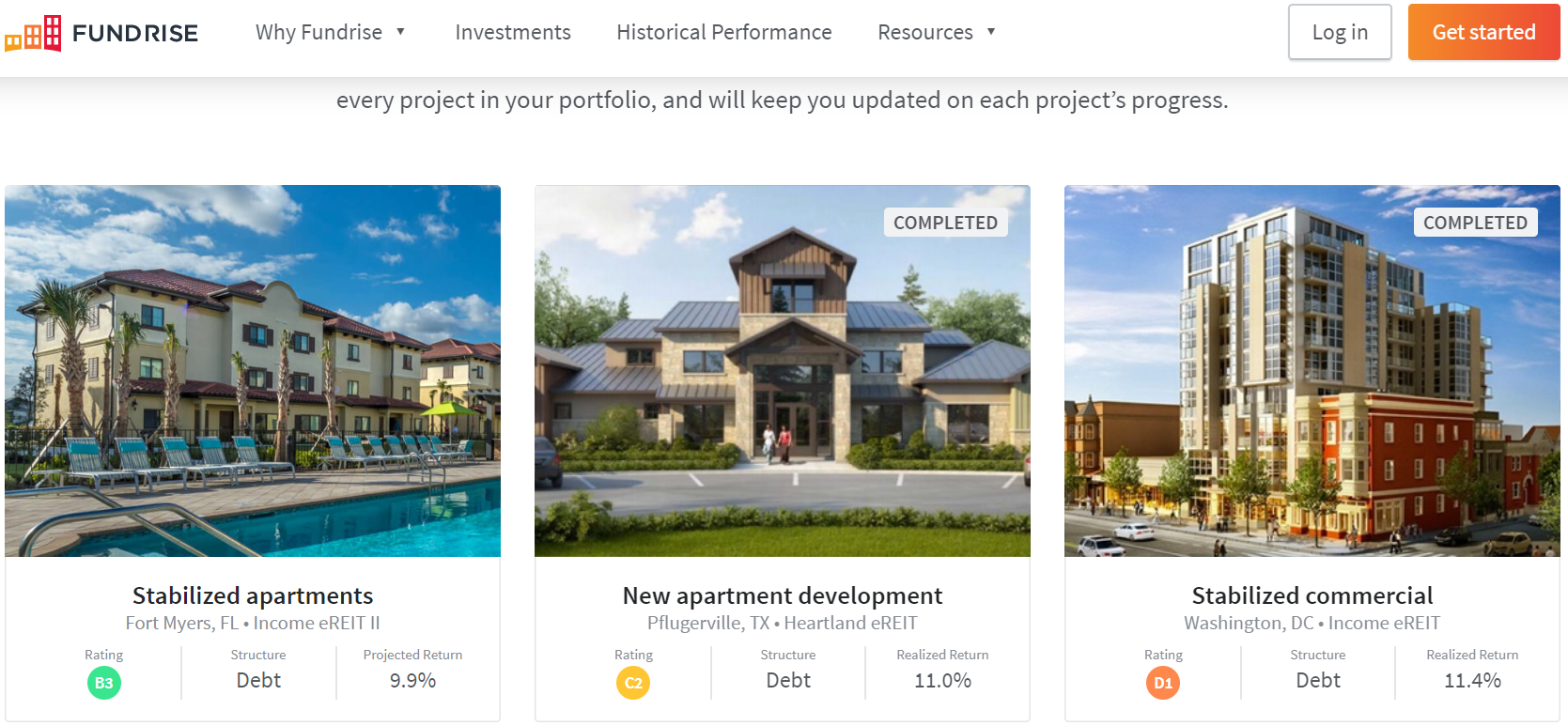The screenshot displays a webpage from the "Fundrise" website, showcasing a detailed view of three different real estate projects. At the top of the page, the "Fundrise" logo is prominently featured next to three small building icons, alongside navigational tabs labeled "Why Invest?", "Why Fundrise?", "Investments," "Historical Performance," and "Resources." To the right, there are buttons for "Login" and "Get Started," the latter highlighted with an orange border.

Central to the image are three property visuals, representing different stages and types of real estate investments. The first is labeled as a "Stabilized Apartment," the second as a "New Apartment Development," and the third as a "Stabilized Commercial" property. Two of these projects are marked as completed, while the third appears to be still in progress. Beneath each property image, detailed information is provided, including ratings, debt levels, and projected returns. The webpage emphasizes that investors can stay updated on the progress of each project in their portfolio.